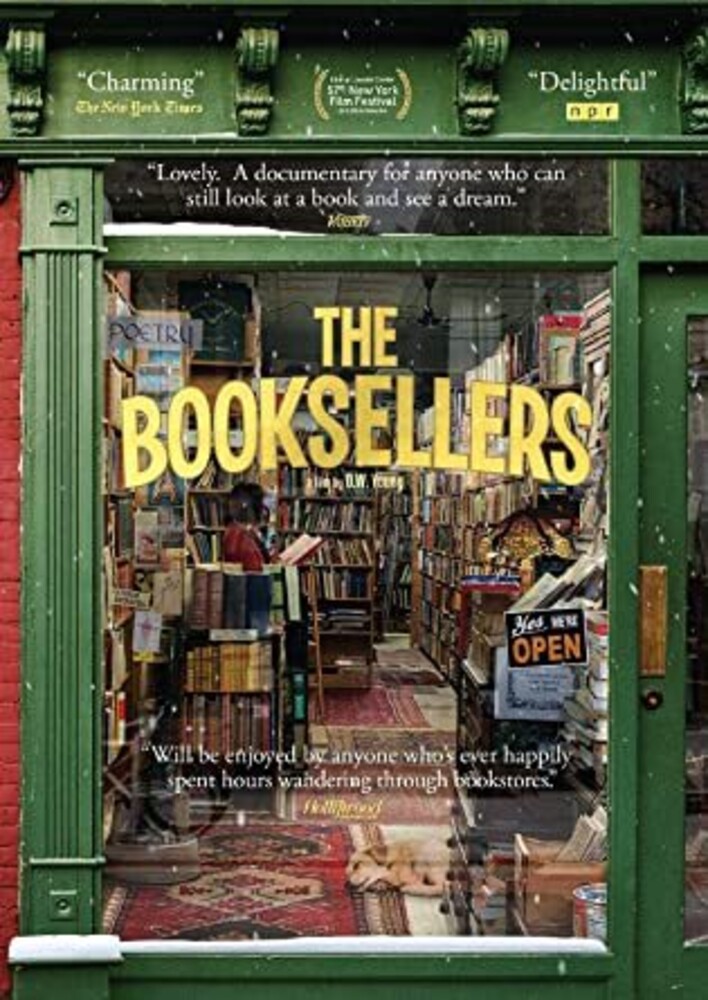This is a detailed photographic image of the storefront of a bookstore, prominently displayed on what appears to be a movie poster for a film titled "The Booksellers." The setting is an outdoor city street during daytime, capturing the view from the perspective of someone standing directly in front of the store. 

The storefront is characterized by its green framing, including both the large window and the door adjacent to it. The substantial glass window features the title "The Booksellers" in gold lettering, with the tagline above it stating, "lovely, a documentary for anyone who can still look at a book and see a dream," attributed to Variety. A sign within the window proclaims, "Yes, we're open," printed in a contrasting black background with white and orange text.

Beneath the main title, another quote reads, "Will be enjoyed by anyone who’s ever happily spent hours wandering through bookstores," although the source of this recommendation is illegible. Above the title, there are notable reviews: NPR calls the film "delightful," and the New York Times labels it "charming." Additionally, it's mentioned that the film was featured at the 57th New York Film Festival.

Through the clear pane of glass, the cozy interior of the bookstore is visible, filled with wall-to-wall, floor-to-ceiling bookshelves, oriental rugs, and a person in a red shirt engrossed in a book. The green door next to the window has a brass hand panel, adding to the store's vintage charm. The scene evokes a sense of nostalgia and wonder, inviting passersby to immerse themselves in the world of books.